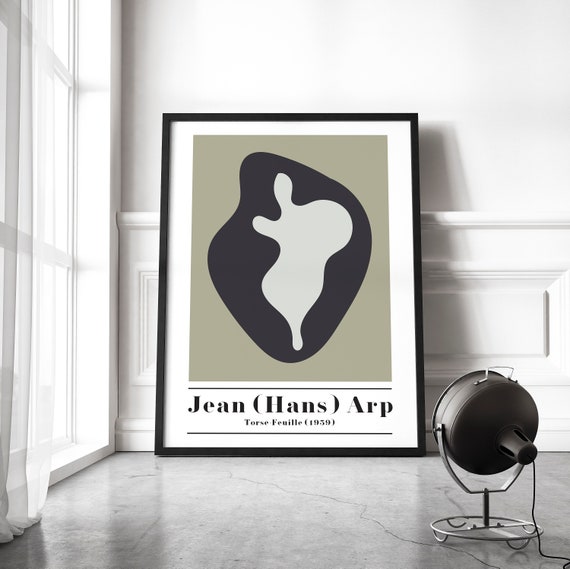This photograph captures an art print leaning against a white wall with white molding up to about three feet high. The image is framed in black plastic with a white border surrounding a gray square. Central to the composition is a black, amoeba-like shape that contains a white, amoeba-like form with two tentacle-like extensions at the bottom. Below the image, on the white border, is text that reads "Jean (Hans) Arp," followed by "Torse-Fenille (1959)." The scene is bathed in natural light from a full-height window with white curtains to the left, and a small spotlight in the bottom right suggests the potential for evening illumination. The floor appears to be light-colored, possibly hardwood or concrete.